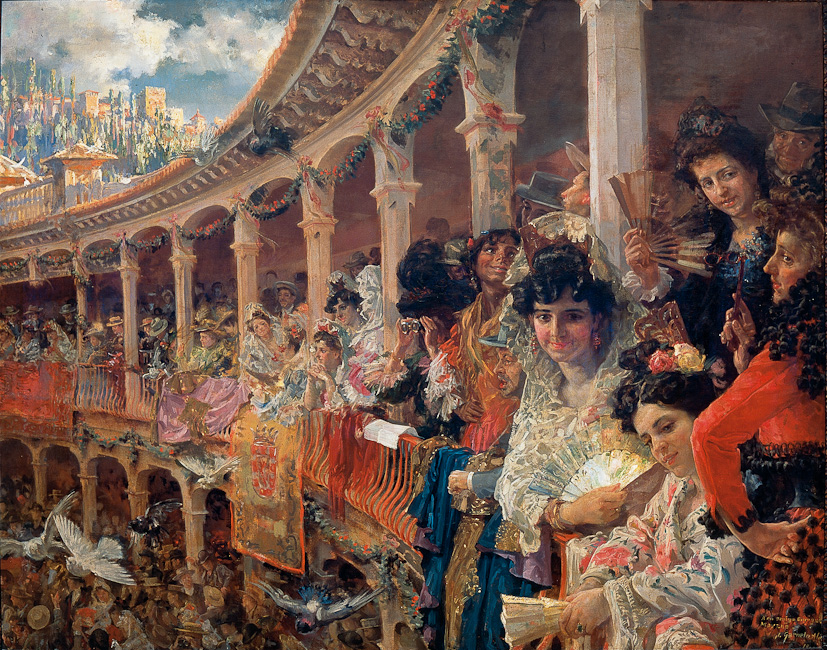The painting portrays an opulent outdoor theater scene from the 1800s, capturing a moment of vibrant social interaction among the aristocracy. The upper level of this amphitheater is lined with elegantly dressed women in vibrant gowns, their ensembles accented with fans. They lean over the ornate railings, engaged in animated conversation, smiles brightening their faces. The women are the focal point, though a few men can be seen scattered throughout, with one particularly noticeable man in the top right corner, wearing a hat and looking directly at the viewer.

This upper tier, divided by beautifully decorated columns adorned with green garlands, stretches from one side to the other, and is festooned with banners and pink tapestries. The amphitheater also has multiple lower levels teeming with people, adding to the bustling atmosphere. White and black doves flit gracefully inside the theater, adding to the sense of anticipation.

In the background on the left side, the open-air design allows a glimpse of a distant cityscape with tall stone buildings, evocative of ancient architectural styles, against a sky filled with puffy white clouds. The painting's vibrant color palette features reds, blacks, whites, and beiges, encapsulating the grandeur and festivity of the moment. The artist's logo is discreetly placed at the bottom right, leaving the intricate and lively scene as the main focus.